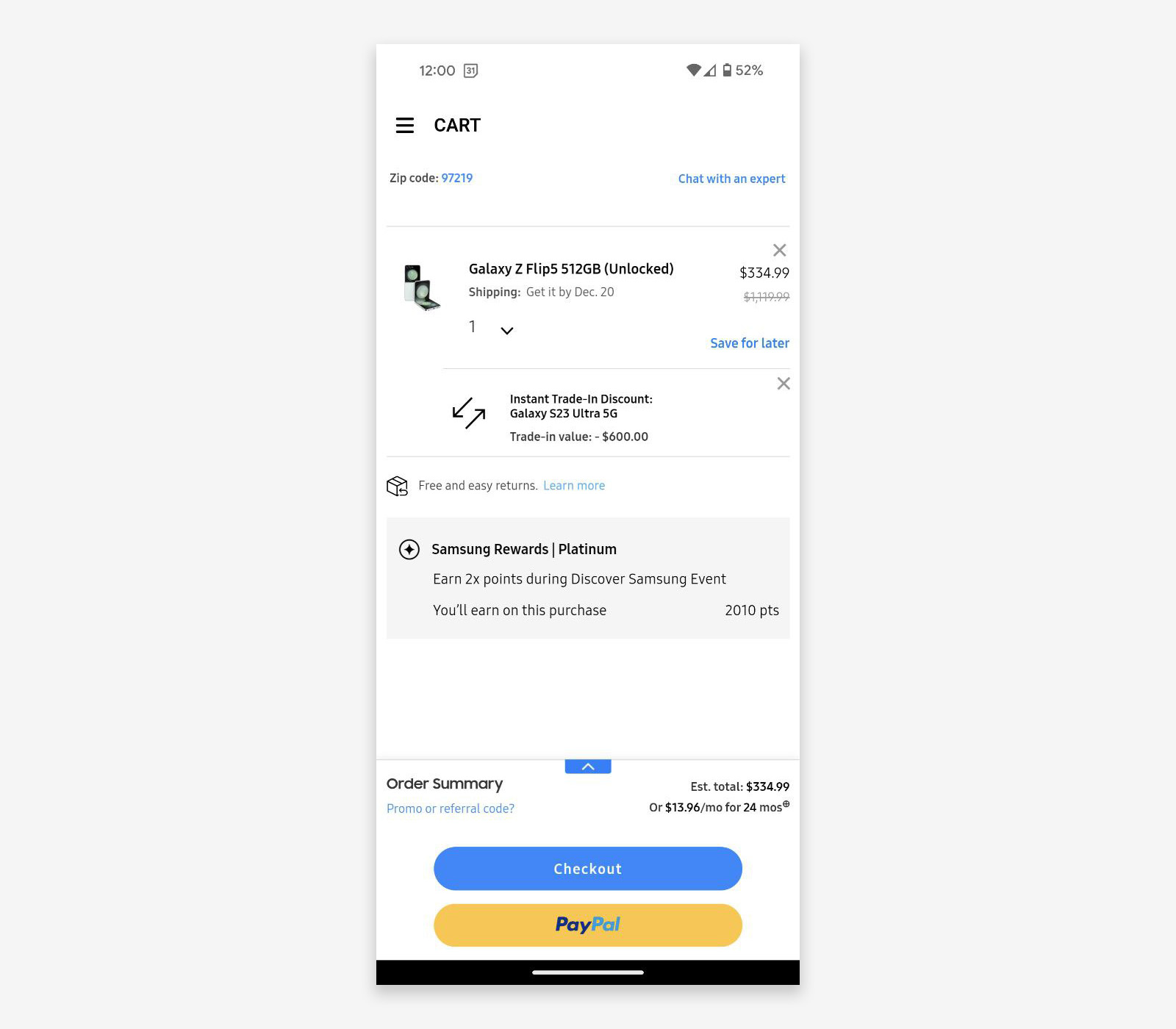This is a vertically oriented image featuring a smartphone screen overlay on a plain gray background. The background is untextured and lacks dimension, appearing as a simple gray canvas. The smartphone screen displayed in the image shows various elements from a shopping application.

At the top left corner, the current time is displayed as 12:00, while on the top right there are icons for Wi-Fi connectivity, battery life at 52%, and a location indicator. The top left also features three horizontal lines, serving as a menu for more options, followed by the word "CART" in bold, uppercase letters. Directly below that, a blue-highlighted zip code "97219" is visible, and adjacent to it, a link for “chat with an expert.”

A horizontal line separates the header with the main content, which begins with an image and description of the Samsung Galaxy Z Flip (512GB, Unlocked). It details the shipping information, promising delivery by December 20th. The quantity is set to one, with an option to remove the item by pressing an 'X,' and the discounted price is prominently displayed at $334.99, down from $1,199. Additionally, there is a "save for later" option in blue text. 

Other interactive elements include bidirectional arrows representing the "Instant Trade-In Discount" for trading in a Galaxy S23 Ultra 5G, valued at $600, along with an option to remove this offer via another 'X'. An icon indicates "free and easy returns," and a blue "learn more" button provides further information.

A gray rectangular box highlights the "Samsung Rewards Platinum" program, promoting a two-times points bonus during the Discovery Samsung event, mentioning that the user will earn 2,010 points on this purchase.

At the bottom of the screen, the order summary section is presented, offering fields for a promo or referral code. There are also two prominent checkout options: a blue button for standard checkout and a yellow button for PayPal.